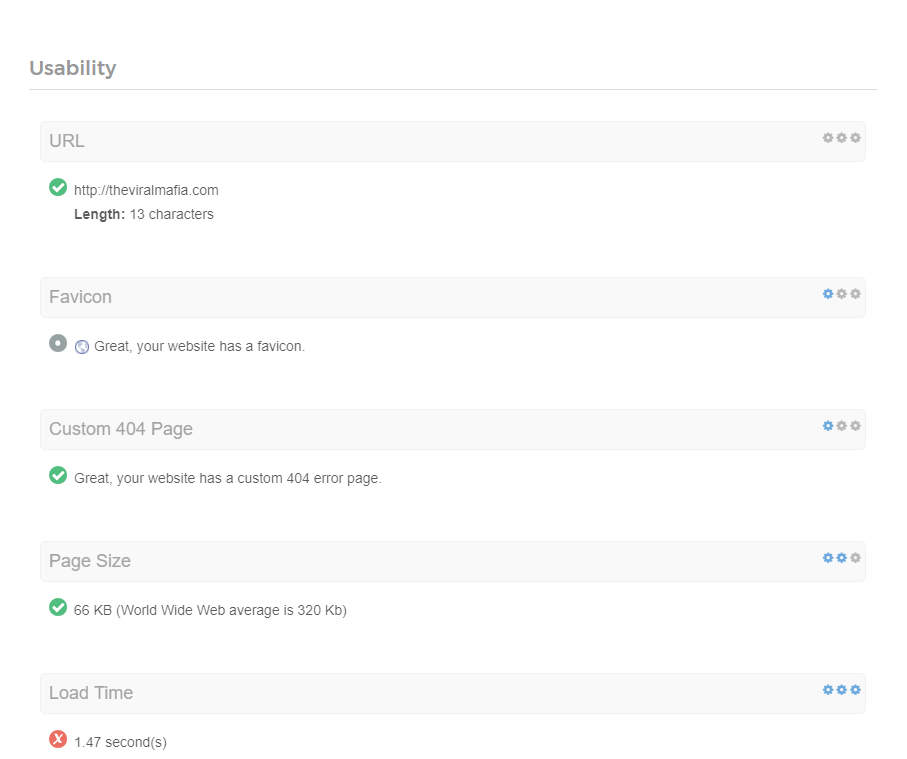Screenshot of a Website Usability Checklist:

The image displays a usability checklist for a website, likely belonging to an individual evaluating their website’s overall performance and user-friendliness. Here are the key details noted in the screenshot:

1. **URL**: 
   - **Status**: Verified (indicated by a green checkmark)
   - **URL Address**: http://theviralmafia.com
   - **Length**: Character count specified

2. **Favicon**:
   - **Status**: Present (marked as 'Great')
   - **Explanation**: The website has a favicon, though the term seems unfamiliar to the observer (represented by 1 out of 3 gears on the usability scale).

3. **Custom 404 Page**:
   - **Status**: Confirmed (indicated as 'Great')
   - **Details**: The website includes a custom 404 error page, enhancing user experience when a page is not found (represented by 1 out of 3 gears).

4. **Page Size**:
   - **Page Size**: 66 kilobytes
   - **Comparison**: Below the Worldwide Web average of 320 KB (rated with 2 out of 3 gears).

5. **Load Time**:
   - **Load Time**: 1.47 seconds
   - **Indicator**: Poor performance (marked by a red X), suggesting the load speed did not meet the desired criteria despite being the highest rated at 3 out of 3 gears.

Additionally, on the right side of the screenshot, gear icons next to each criterion visually represent the usability score, contributing to a more detailed and organized analysis.

This comprehensive review likely assists the website owner in identifying strengths and areas for improvement, particularly regarding load time and overall efficiency.